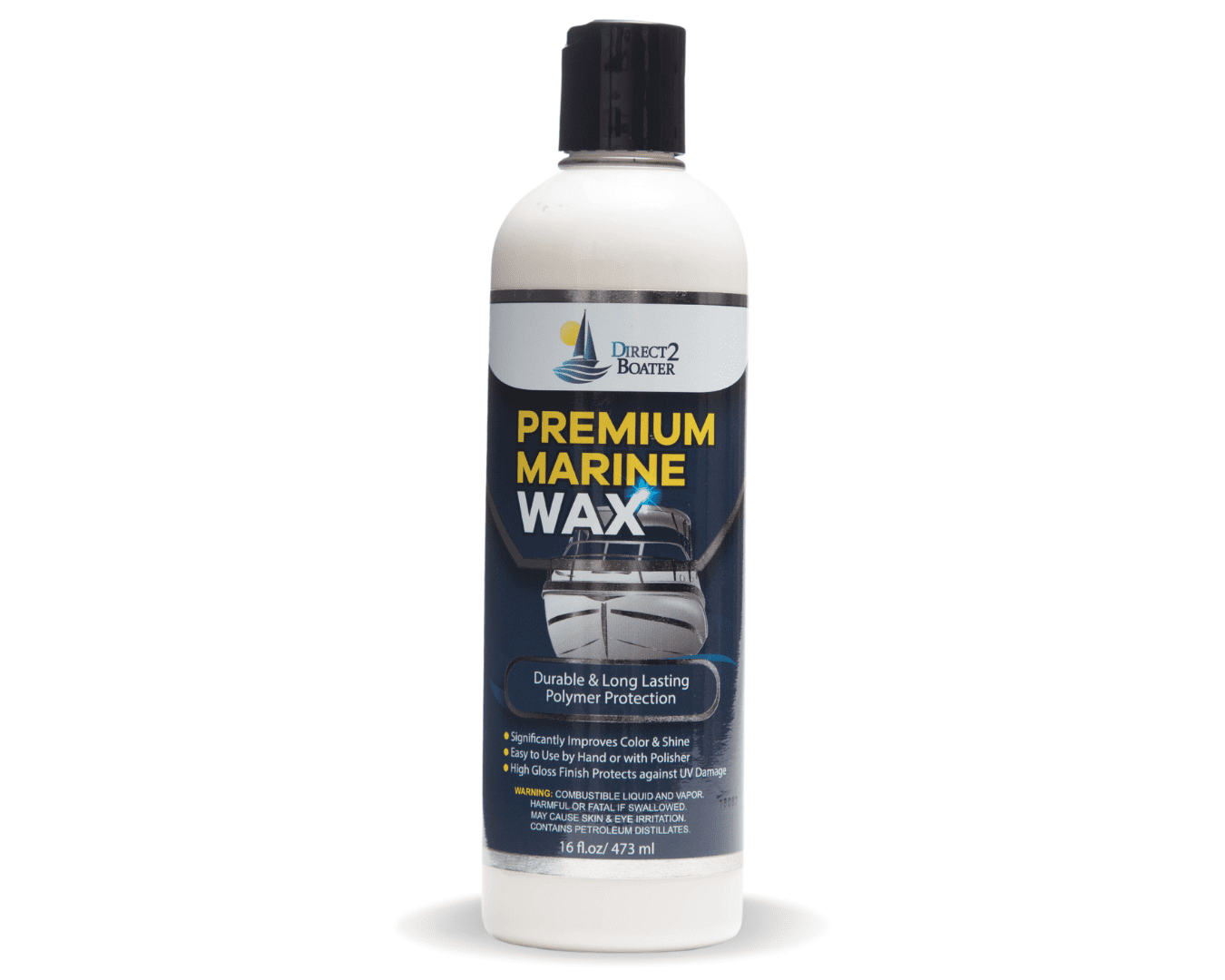This is a detailed photo of a bottle of premium marine wax, featuring a clear plastic or tin-like white bottle with a black cap. The label is predominantly black on top, transitioning to white below. At the top of the label, it reads "Direct to Boater" next to a clip art image depicting a sailboat with sails and a sun, resembling a company logo. Directly beneath this, in yellow, it states "Premium Marine" followed by the word "Wax" in larger white letters. Below these texts, there's an image of the front of a large white yacht set against a blue backdrop with the text "Durable and Long-Lasting Polymer Protection" encased in a black oval. Further down, highlighted by yellow dots, the label explains that the product "Specifically improves color and shine," is "Easy to use by hand or with polisher," and provides a "High-gloss finish, protects against UV damage." At the bottom of the label, there is a warning in yellow text, and the bottle's capacity is noted as 16 fluid ounces (473 milliliters). The image has a shadow but no background, emphasizing the bottle’s colors: a mix of yellow, black, white, and a touch of blue.